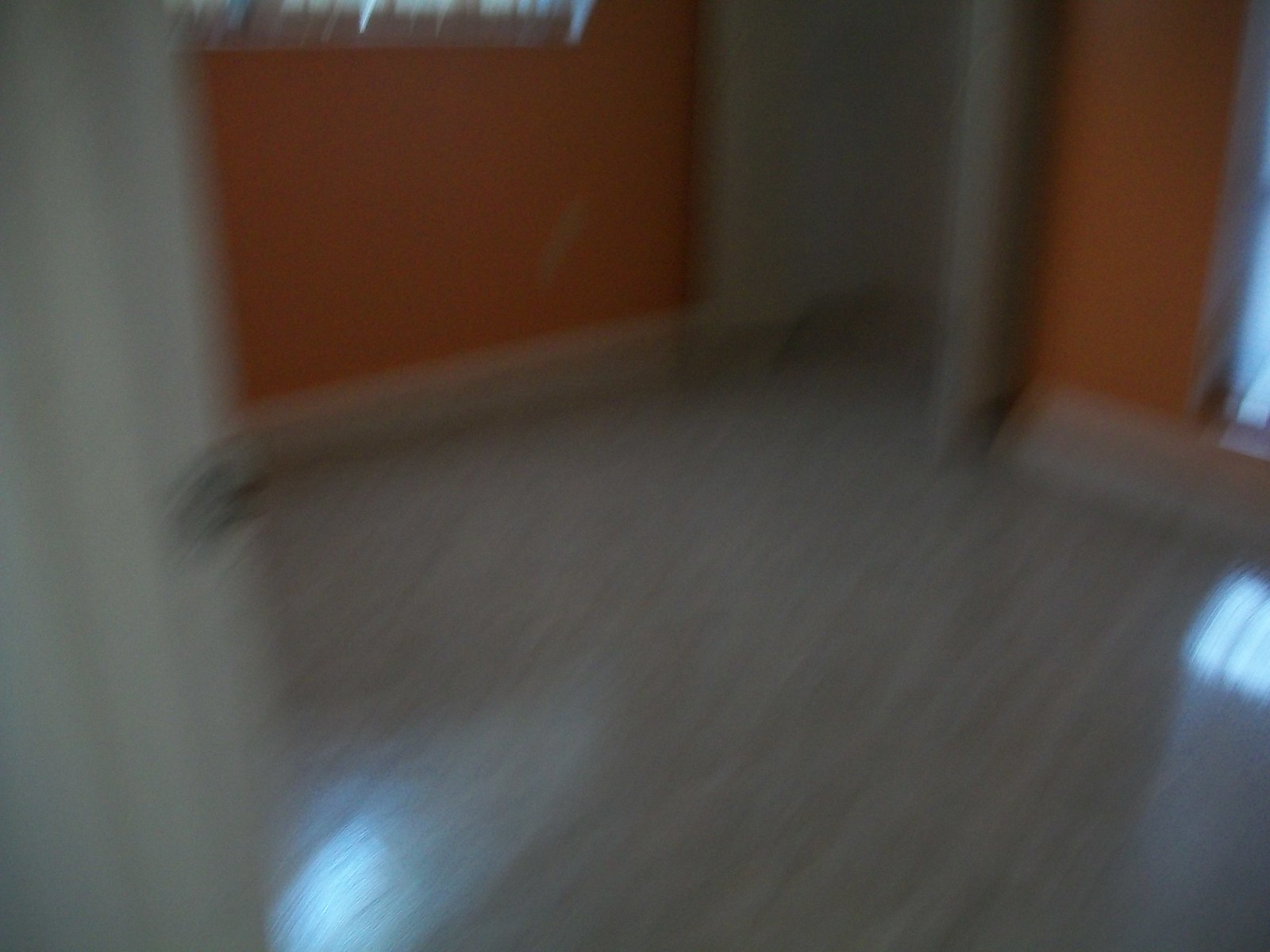The image is slightly blurred but reveals various distinct elements. On the left-hand side, there's a white wall featuring vertical lines. The floor is a light brown wood color and reflects light on both the right and left sides. Brown-colored floorboards run along the base of the walls around the room. At the far end of the image, there's an orange wall situated in the center, extending slightly to the right. Additionally, an orange wall occupies the right-hand side of the frame, allowing light to filter through. Between these two orange walls, there's a brown section that likely represents either a wall or an open door.